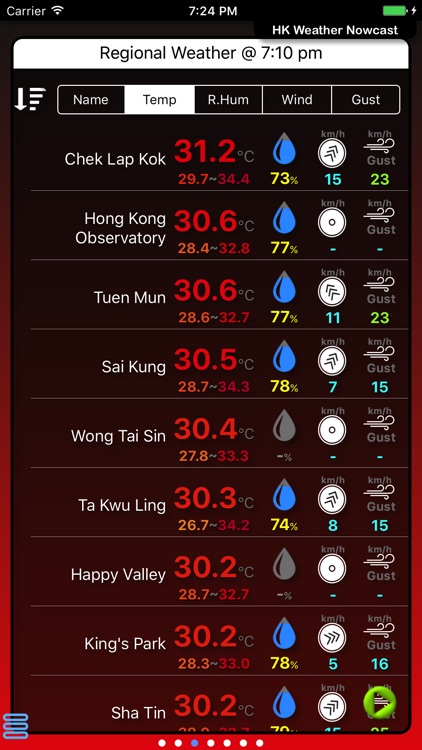In the upper right corner of the image, there's a full green battery icon and the time displayed as 7:24 p.m. Directly below that, a large white rectangle titled "HK Weather Nowcast" shows regional weather information as of 7:10 p.m. Within this rectangle, there are several labeled options: "Name," "Temp" which stands for temperature, "RHUM" indicating humidity, "Wind," and "Gust."

Underneath these options, for Chek Lap Kok, the temperature is listed as 31.2°C, with a 73% chance of rain represented by a blue raindrop icon. Additionally, wind speeds range from 15 to 23, as illustrated by the wind icon.

Other locations displayed include the Hong Kong Observatory, Tuen Mun, Sai Kung, Wong Tai Sin, Tai Koo Ling, Happy Valley, Kings Park, and Sha Tin. The rain probability for these areas varies between 73% and 78%, while wind gusts range from none to speeds between 15 and 23.